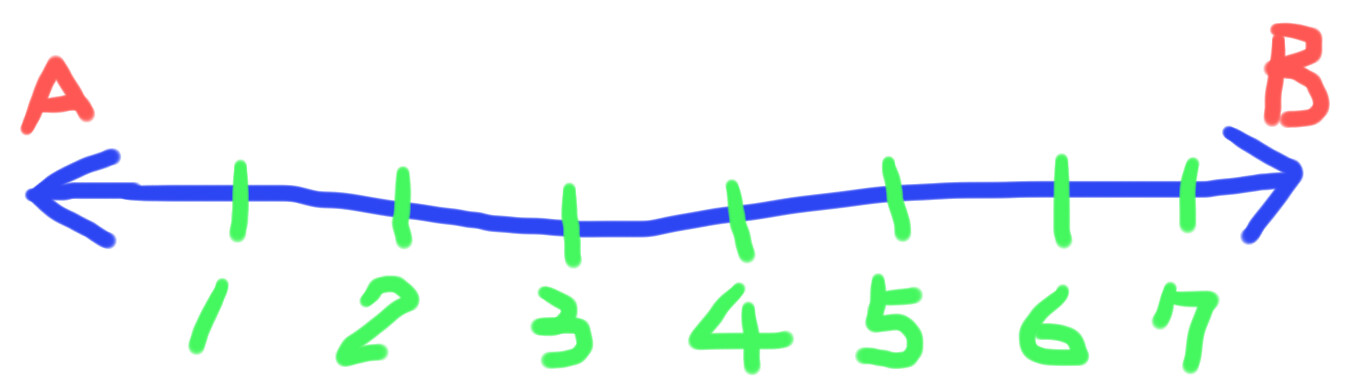This is a freehand drawing on a plain white background, featuring a prominent horizontal blue line that extends unevenly across the image. The line is capped with arrows at both ends, signifying direction. Positioned above the arrow on the left end is a bold, red capital letter "A," while a corresponding blue capital letter "B" is situated above the arrow on the right end. 

Between the arrows, the blue line is intersected by seven bright green horizontal slashes, each unevenly spaced to reflect the freehand nature of the drawing. Beneath each slash is a numeral, sequentially labeled from one to seven. These labels are directly under the slashes, sequentially listing the numbers 1 through 7. The gaps between these labels and their respective slashes vary in length due to the hand-drawn style. Apart from these elements—the line, arrows, letters, slashes, and numbers—the image remains unadorned and simple.